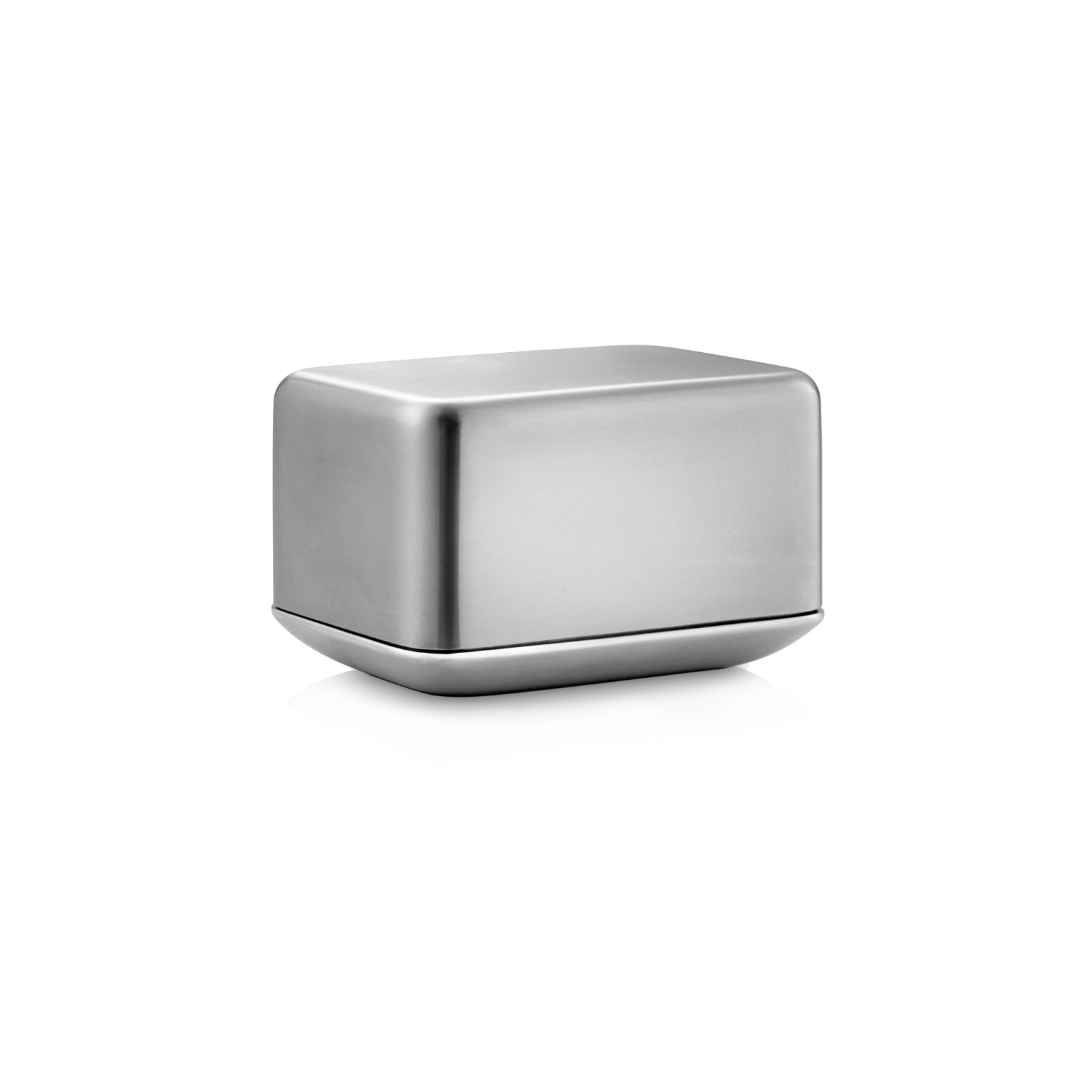The image features a centrally placed, reflective chrome box against a solid white background. The box, which is both rectangular and square-like with rounded edges, is somewhat difficult to identify due to its simplicity and lack of distinctive features such as buttons or slots. It has a bit of a shadow beneath and around the corner facing the viewer, giving it some depth and dimension. The overall look suggests it could be a heavy paperweight or, if slightly smaller, resemble a butter holder used at dinners. The chrome surface adds to its sleek, uncluttered appearance, making the object appear both small and substantial at the same time.